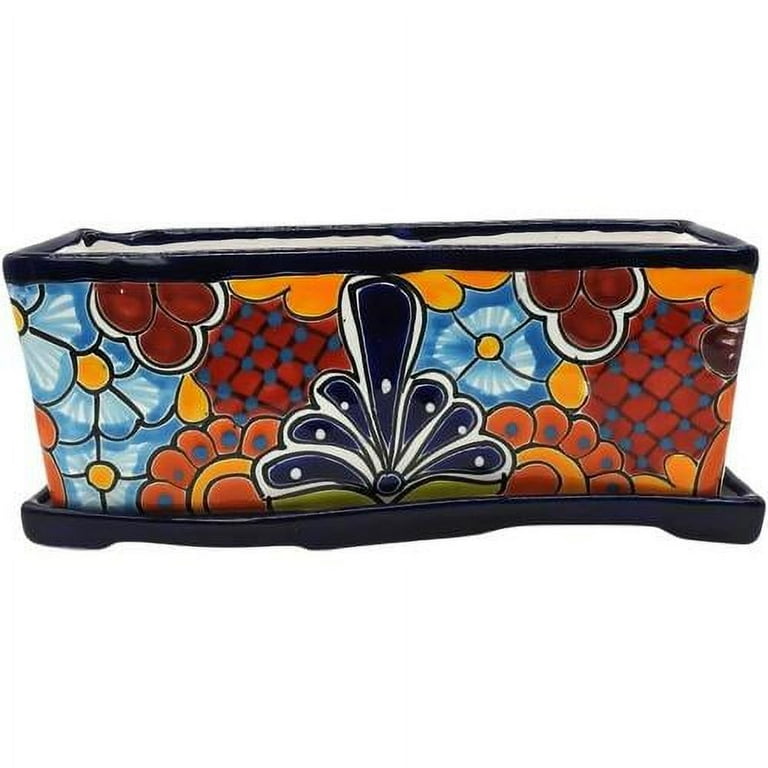The image showcases a vibrantly colored, horizontally rectangular ceramic planter, set against a solid white background. The planter features a black or dark blue base and a matching trim around its top lip. The exterior is adorned with a glossy enamel finish, exhibiting an eclectic floral and decorative pattern. Prominent in the design are blue flowers with yellow centers, interspersed with ball-shaped ornaments in shades of orange, with some featuring light blue dots and others trimmed in yellow. Centrally, there's a striking navy blue exclamation point-like shape, flanked by navy blue feather-like designs with white dots. Additionally, a black peacock feather pattern with a white circle in the middle and white trim adds to the detailed embellishments. The planter appears to also have a drip tray at the base, enhancing its functional aesthetics.